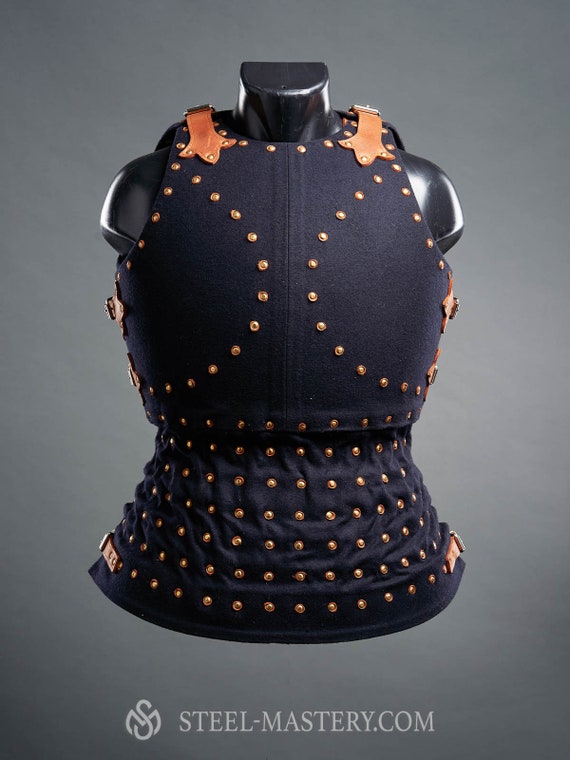The photograph depicts a medieval-style padded armor piece, displayed on a black, armless, headless mannequin against a gray background. The piece, which resembles an undergarment worn beneath exterior armor, features intricate detailing. The armor is primarily made of a navy blue or black fabric material, adorned with numerous golden or bronze rivets. These rivets are arranged in a grid pattern across the lower section covering the stomach area, comprising seven rows. The upper chest area is bordered by rivets outlining the perimeter, with additional circular patterns positioned over the pectoral muscles or ribcage. A central seam runs vertically down the middle of the piece. Tan-colored leather straps, each with a silver buckle, extend over the shoulders. These straps are forked at the ends with three rivets each and buckle below the shoulders. The bottom of the image features the text "steelmastery.com," likely indicating the manufacturer or retailer of the armor.